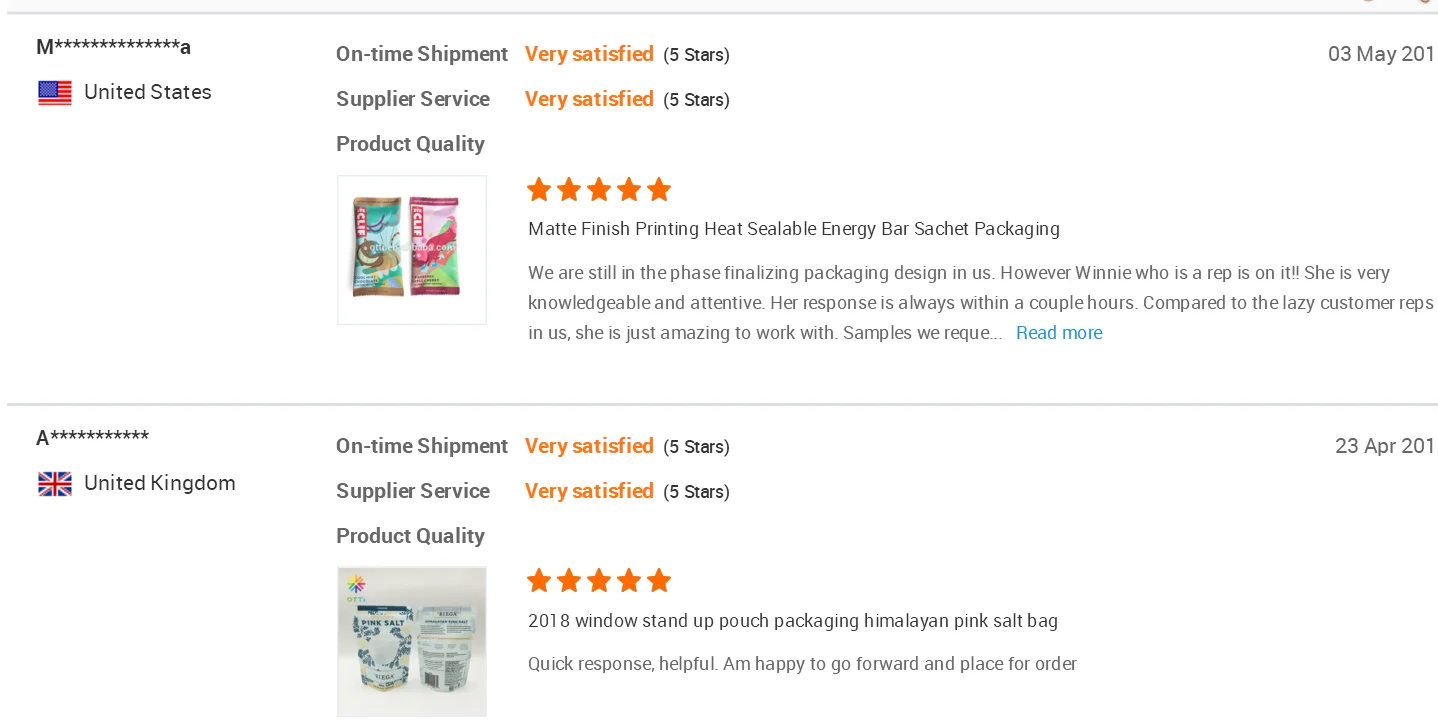The image features a white background with several distinct sections. At the top, there is a small blue box with a dash at the end, followed by a letter "M" adorned with numerous small stars. To the right of this is an "A" and an American flag indicating the United States. Below, the text lists "On-time shipment," "Supplier service," and "Product quality."

Beneath this section is a white box containing two bars wrapped in purple and blue packaging. To the right, there's text in red that reads "Very satisfied" accompanied by five red stars, repeating "Very satisfied" and five stars again. The date "3rd of May 201" is also mentioned, presumably meant to read "3rd of May 2021." It continues with the phrases "Matte finish printing," "Heat sealable energy bar," and "Sachet packaging." The text explains that the packaging design is in the finalization phase in the U.S., with a representative named Winnie described as knowledgeable, attentive, and quick to respond, in contrast to other customer reps. It concludes with "Samples we require. Read more."

A thick blue line separates this section from the next. Here, a large "A" with numerous stars is paired with a British flag indicating the United Kingdom. Similar to the previous section, it lists "On-time shipment," "Supplied services," and "Product quality." There is a small square with an image of two products and a circle featuring red, yellow, and blue colors. To the right, the text reads "Very satisfied" with five red stars twice, followed by the date "23rd of April 201," likely "23rd of April 2021." It mentions "2018 window stand-up pouch packaging," "Himalayan pink salt bag," and concludes with "Quick response, helpful. I'm happy to go forward and place the order."